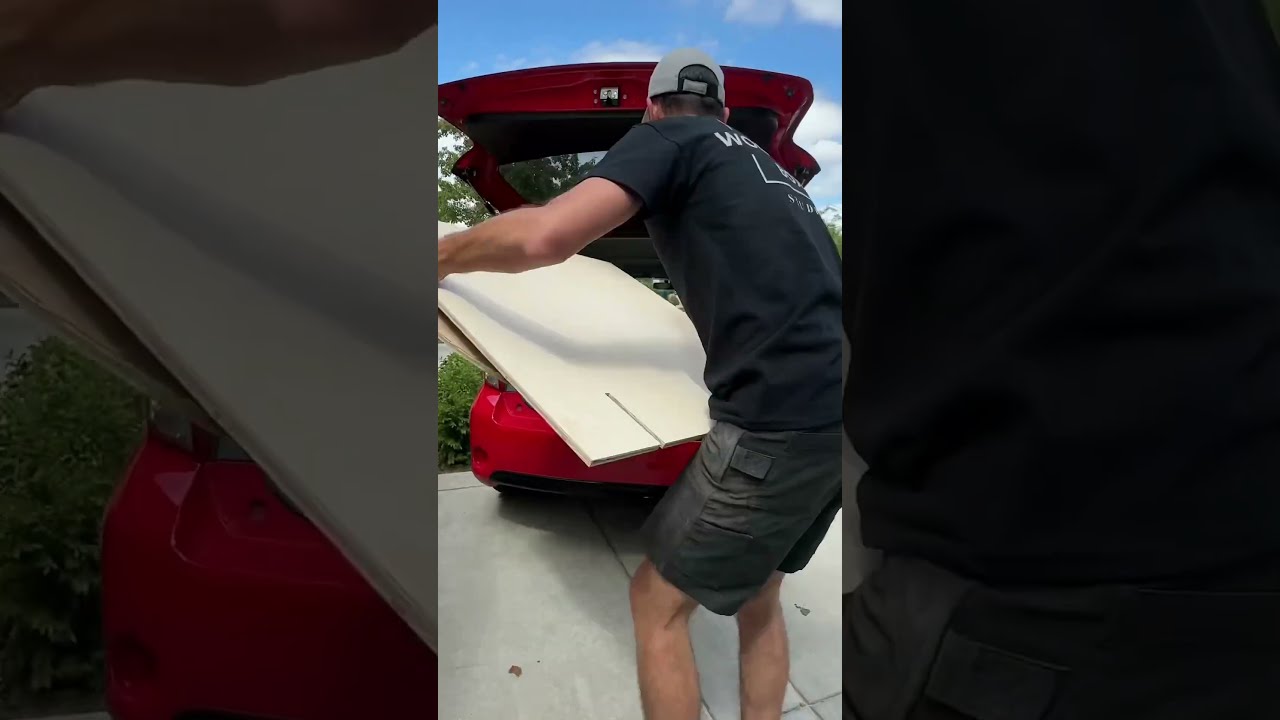In this vertical image, which resembles a screen grab from a video, a young man is seen from behind, his face obscured. His build suggests he is in his 30s. He is dressed in a black t-shirt, dark gray shorts, and a gray baseball cap. The man is slightly hunched over, appearing to load or unload large white boards or construction sheeting from the open trunk of a red hatchback vehicle. The scene is set on a gray concrete surface, likely a driveway, with green shrubbery visible to the left. At the top of the image, the bright blue sky is dotted with light clouds, indicating daytime. The car's tires and license plate are out of view, and there are no other people present in this scene.